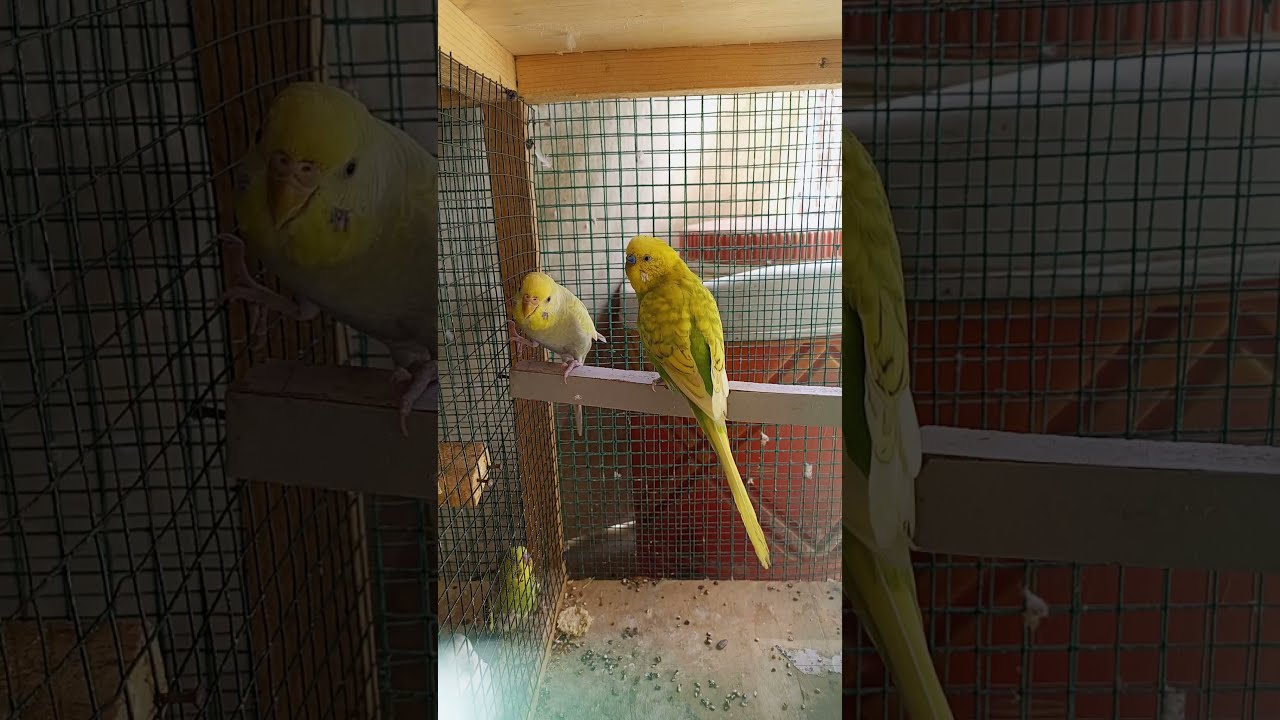In the center of this detailed photograph, we observe three vibrant parakeets inside a pen. Two parakeets are perched together on a brown-painted, wooden beam resembling a 2x2 from Home Depot. These two are positioned centrally within the pen and are framed by the surrounding structure. The first parakeet, primarily yellow with green accents, stands with its back turned towards us, displaying its full yellow feathered wings and tail, while it peeks over its shoulder. The other, positioned to the left, has a grayish body with a yellow head and maintains its grip on the perch with one leg while holding on to the wire mesh with the other. 

Below them, on the bottom of the pen, sits a third parakeet, predominantly green with a yellow face, gazing up at the two perched above. The pen, approximately two feet tall, is constructed with wooden beams and wrapped in small square wire mesh that is green in color, resembling chicken wire, providing a secure enclosure.

Additionally, the photograph includes split-screen close-ups: on the left, a shaded, up-close view of the gray and yellow parakeet, and on the right, a highlighted close-up of the yellow and green parakeet’s back. The bottom of the pen is littered with bird pellets, adding to the detailed and textured environment captured in this image.